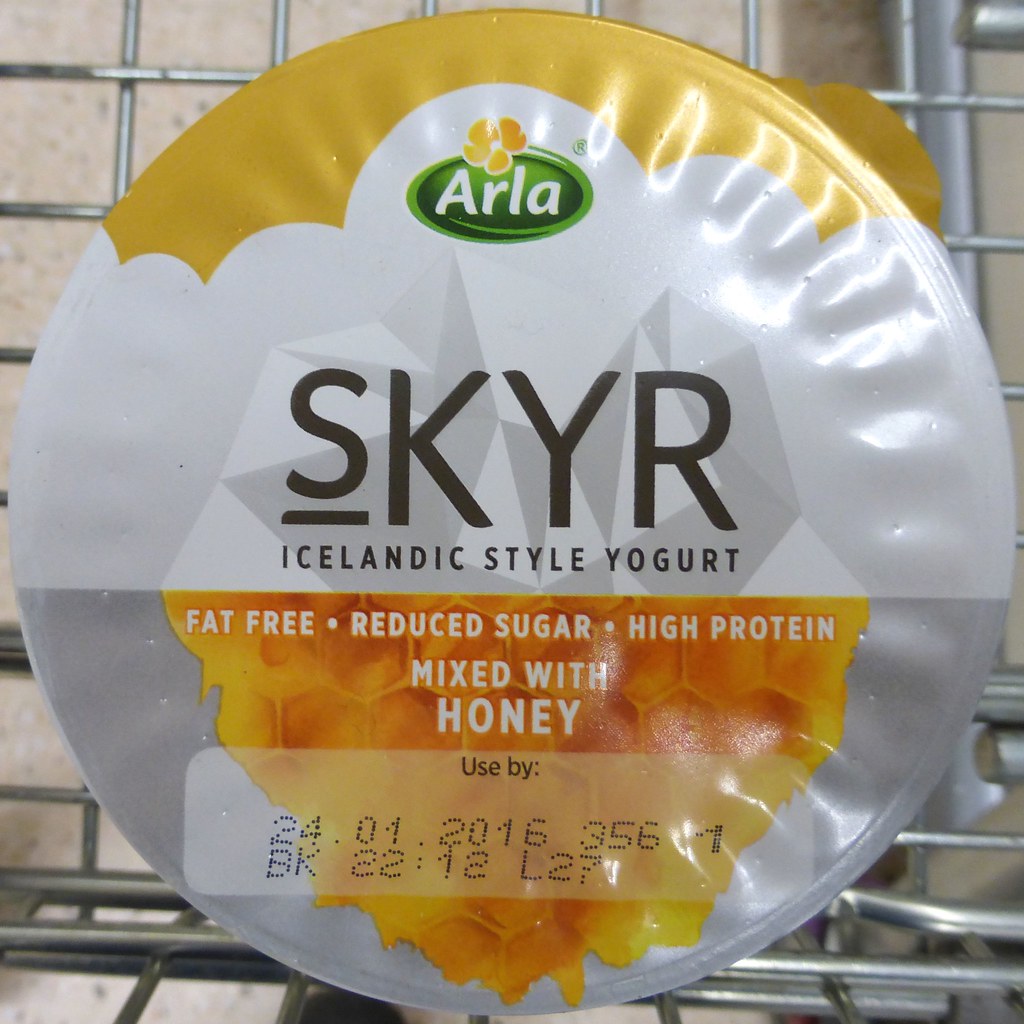The image depicts the top of an Arla brand yogurt container, named Skyer, positioned on a metal grate, likely from a shopping cart. The lid features a combination of silver, white, and gray hues, with a prominent yellow streak across the top. Centrally, there's a green logo with white lettering spelling "ARLA" beneath a golden petaled flower design. Directly below, the product name "SKYR" is displayed in large black letters against a white background, with "Icelandic Style Yogurt" written underneath in smaller letters. The lower third of the lid showcases detailed product information — "fat-free, reduced sugar, high protein, mixed with honey" — in white text on a honey-colored, honeycomb-patterned background, giving a textured visual effect. The use-by date is clearly marked as January 24, 2016, with additional product codes. The lid also has an image of honey that appears to be dripping off, adding to the visual appeal.